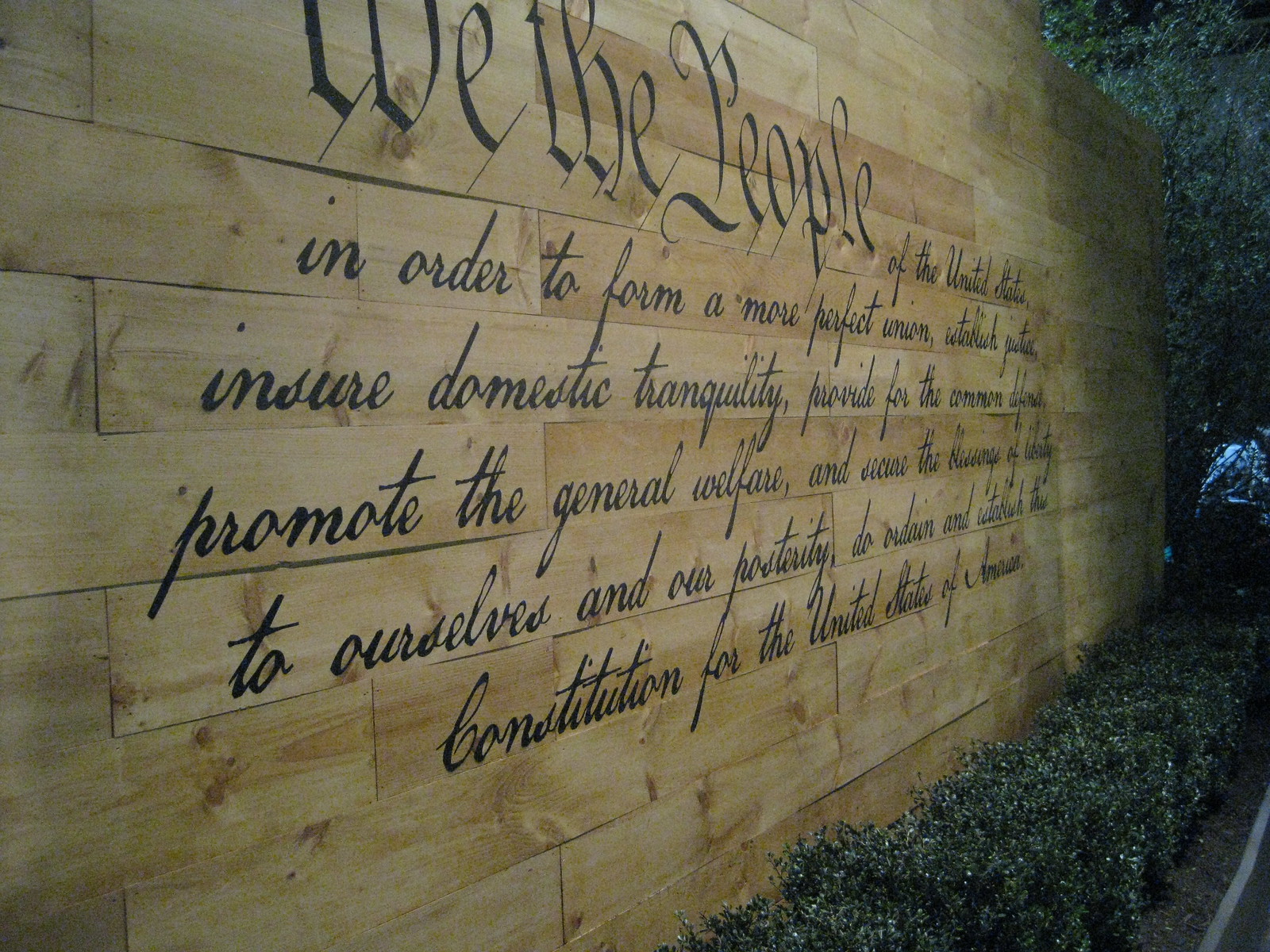This full-color nighttime photograph depicts an outdoor scene featuring a prominent wooden sign with a partial quote from the United States Constitution. The sign is positioned diagonally in the center of the image, and it displays the text in black cursive, replicating the original handwriting of the Constitution. The visible portion of the quote reads: "We the People of the United States, in Order to form a more perfect Union, establish … ensure domestic Tranquility, provide for the … promote the General Welfare, and … to ourselves and our Posterity, do ordain and establish this Constitution for the United States of America." Surrounding the sign, the far right side of the image reveals a paved area with a white dividing line, accompanied by small plants, patches of dirt, and some bushes. In the upper right corner, trees are visible against the night sky, providing a backdrop to this tranquil, historical outdoor setting. The color palette includes shades of tan, black, green, gray, white, and hints of light blue.